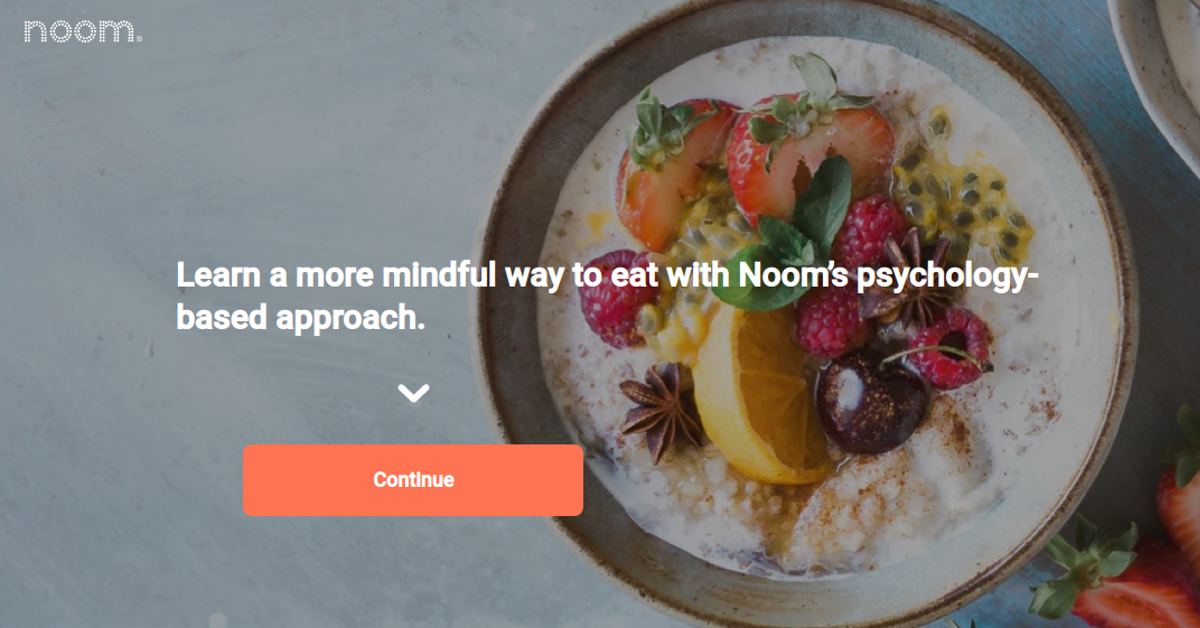This is a landscape-oriented screenshot from the Noom app, a platform focused on health and dieting. At the top left corner, the Noom logo is displayed in lowercase letters with a distinctive polka dot pattern, followed by a period. The backdrop of the image captures a picturesque scene reminiscent of a neatly set dining table.

In the foreground, there is a visually appealing bowl with a white interior and a brown rim, filled with what appears to be a rich-textured food item that could be oatmeal or yogurt. The bowl is garnished with an assortment of fresh fruits, including strawberries, lemons, various berries, and a black cherry, enhancing its visual appeal. Slightly behind this main bowl, another bowl is partially visible, adding depth to the image. Two strawberries are positioned at the bottom of the frame, further contributing to the vibrant arrangement.

At the center of the image, white text reads: "Learn a more mindful way to eat with Noom's psychology-based approach," encouraging a thoughtful approach to eating. Below this text is a downward arrow and a prominent, rectangular, rounded-edged button in a pinkish-orange hue, labeled "Continue." This button suggests that clicking it would allow users to log into the Noom site and explore insights on mindful eating and improving eating habits. The image effectively conveys Noom's focus on the intersection of food and psychology, inviting users to begin their journey towards healthier eating habits.